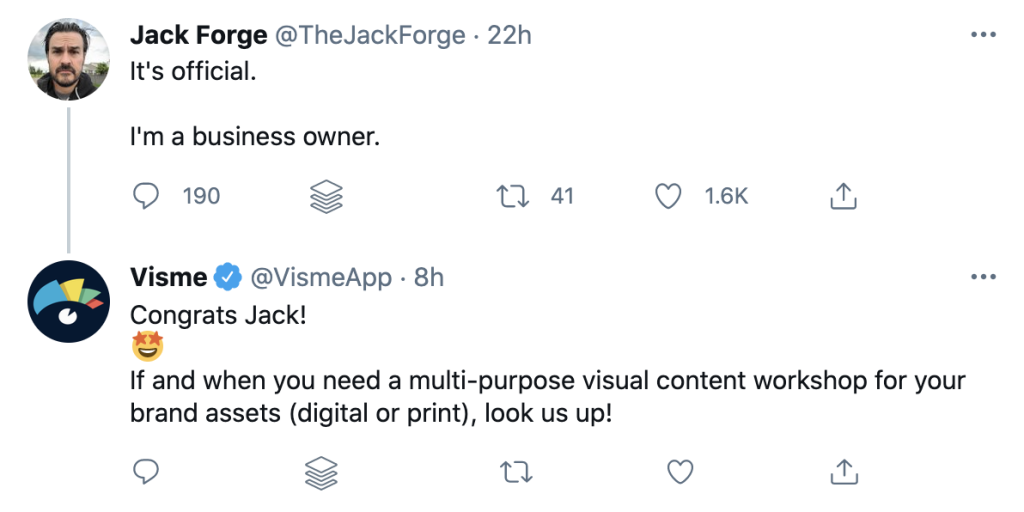**Screenshot Description:**

The screenshot captures a Twitter interaction between two users. The primary tweet is from Jack Forge (@JackForge), posted 22 hours ago, featuring his profile picture in a small circle. The tweet reads: "It's official, I'm a business owner." It has garnered significant engagement with 190 comments, 41 retweets, and 1,600 likes. 

Below Jack's tweet, there's a reply from VisMe (@VisMeApp), posted 8 hours ago, with a profile picture displaying a circle with a blue, yellow, green, and red page of paper. Their response states: "Congrats, Jack! 😊 If and when you need a multipurpose visual content workshop for your brand assets (digital or print), look us up!"